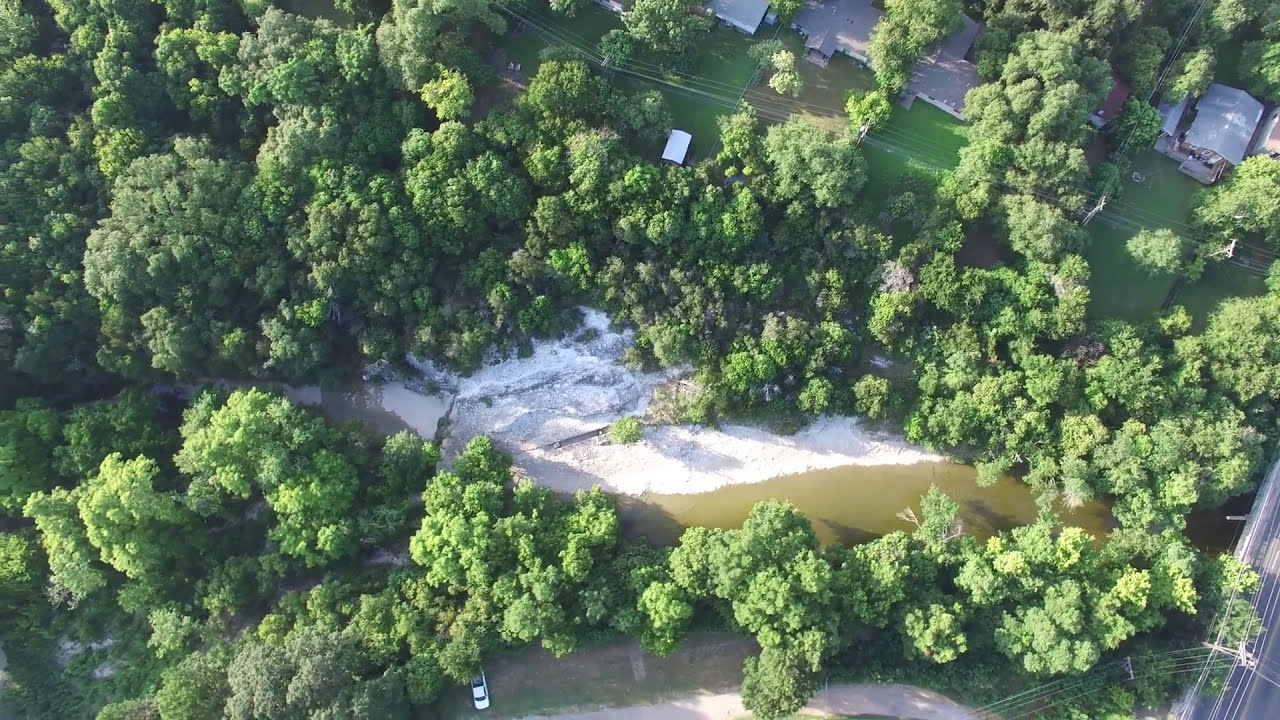This aerial photograph depicts a residential neighborhood characterized by a mix of natural and human-made elements. At the heart of the image lies a central water feature, which could be a stream or a small pond, its brownish tint suggesting recent flooding or sediment-rich waters. Surrounding this body of water is a sandy or possibly snowy area, though the exact nature of this white expanse is ambiguous due to the shadows cast across the scene. 

In the upper right corner, several houses with gray roofs are visible, contrasting with the lush, green, bushy trees that dominate the landscape. The lower right corner of the image features a dirt road, where a white car is parked. Additionally, power lines are seen cutting through the frame at both the top and the lower right, adding to the suburban feel of the setting. The brightness of the day creates sharp shadows, further complicating the identification of some elements but contributing to the scene's overall clarity and detail.